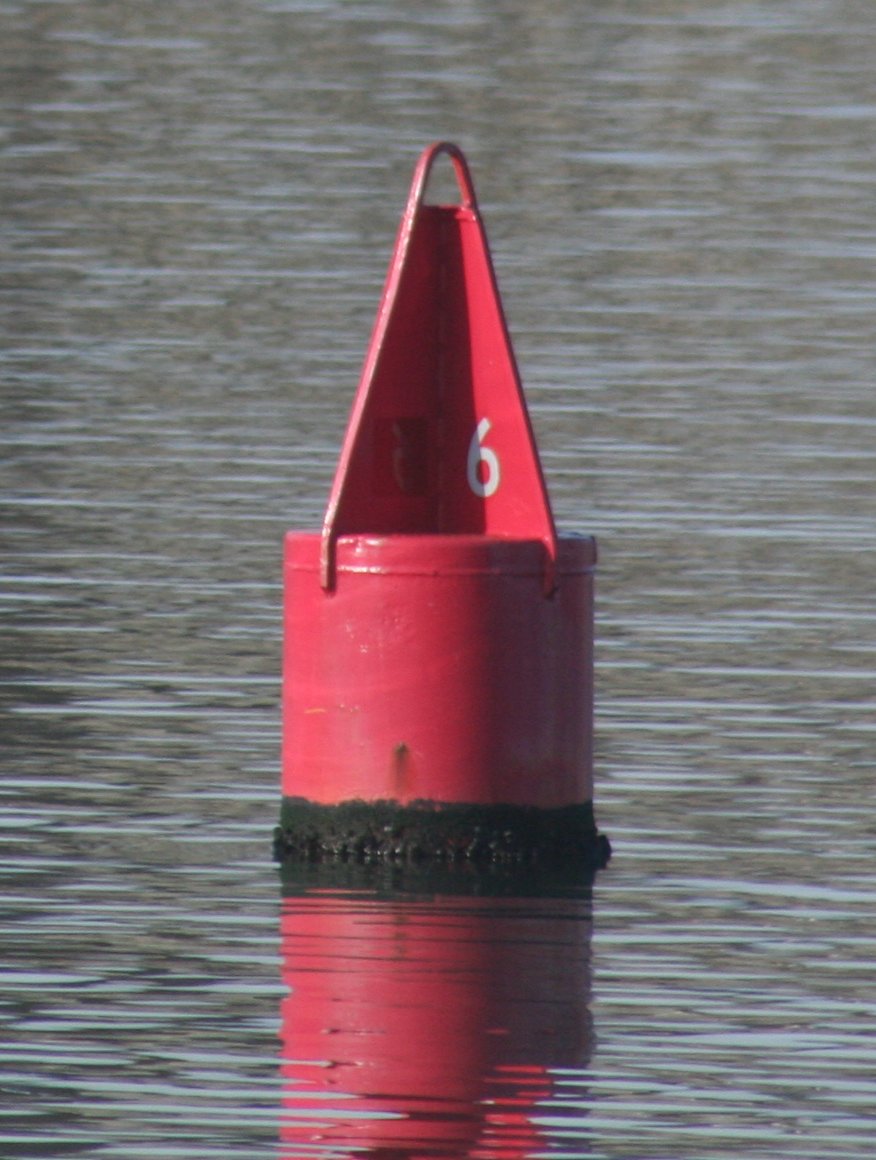This image captures an isolated buoy floating in what appears to be an expansive body of water, likely a lake given the descriptions of its size and distance from any visible shorelines. The buoy is a striking bright red color, made of what seems to be steel or a similar metal. It stands prominently in the water, its cylindrical body giving way to a conical top featuring a large number "6" painted in white. The top also includes a triangular fin-like panel with a loop, creating a distinct silhouette against the backdrop of the open water. Around the base of the buoy, where it meets the water, it appears darker, possibly due to black paint, barnacles, or rust accumulation, giving it a textured and weathered look. The water itself is not very clear, adding to the buoy's rugged appearance in this serene aquatic setting.